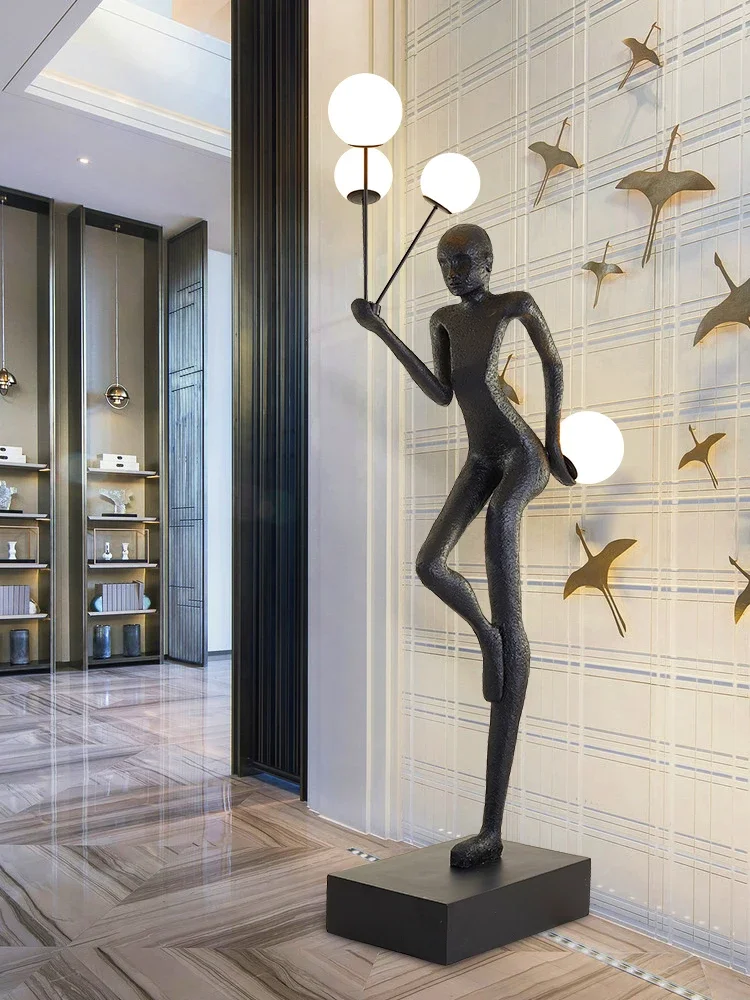In the picture, we see a captivating museum installation featuring a tall, elongated sculpture of a person. This slender, dark gray metal figure stands with twisted, slightly warped proportions. It balances delicately on a black box, its left leg straight and its right leg bent and braced against the left knee. The sculpture’s right hand extends forward, clutching three vertical metal rods topped with glowing white orbs, reminiscent of lollipops. Meanwhile, the left hand reaches behind to cradle another glowing orb against the figure’s buttocks. The background highlights a serene white wall adorned with nine golden silhouettes of cranes in flight, evoking a sense of graceful movement. The scene is set on a reflective brown floor with neatly aligned square planks. On the left side, two display cases filled with historical items add context and depth to the museum setting.